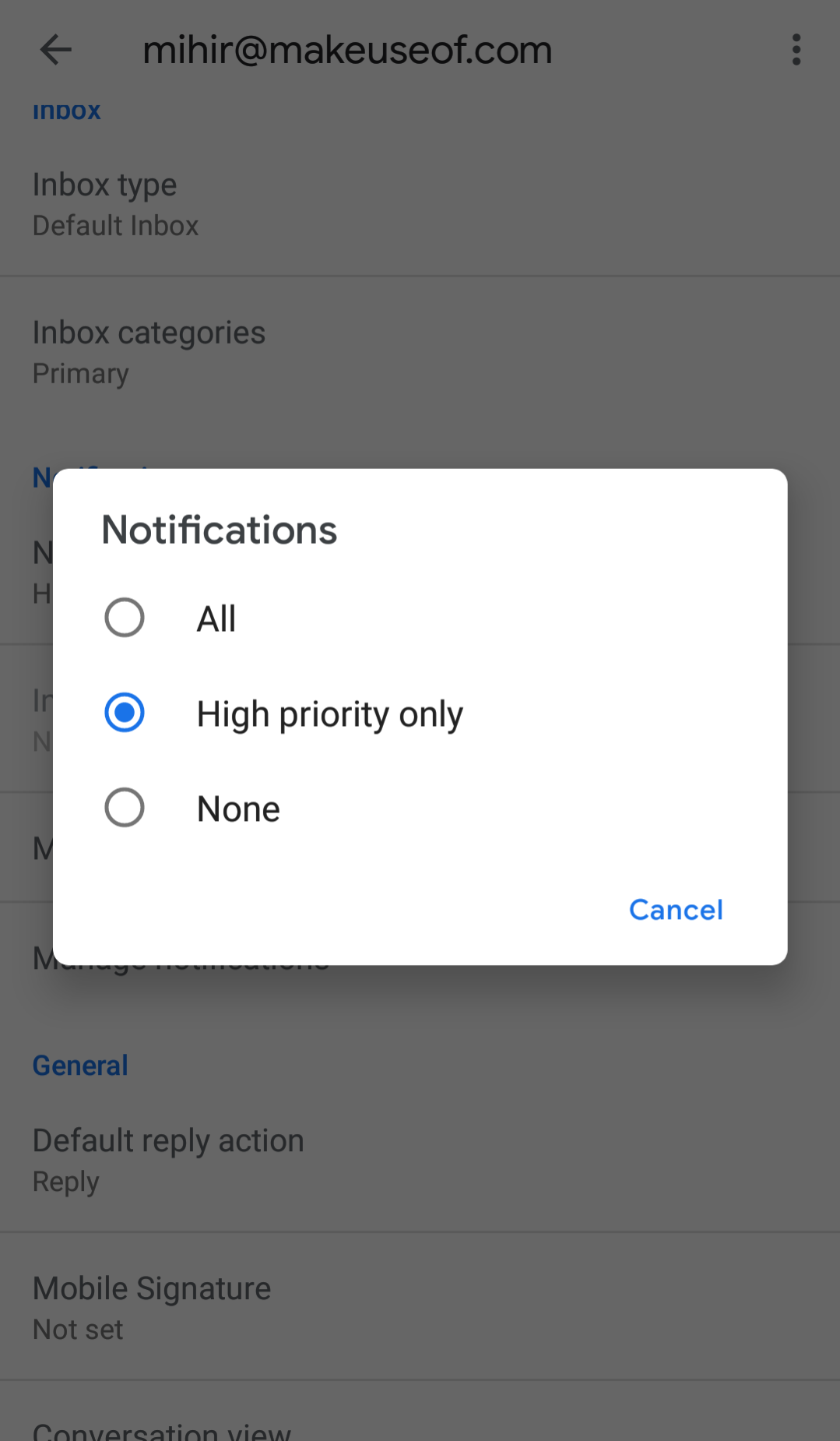**Caption:**

A mobile phone screen displaying a notification settings pop-up. The pop-up, a white rectangle, prominently features the title "Notifications" at the top, followed by three option circles labeled "All," "High Priority Only," and "None." The "High Priority Only" option is selected, indicated by a blue-filled circle. In the lower-right corner of the pop-up, two buttons read "Cancel" and "Blueprint."

The pop-up overlays a partially visible email settings screen from "MIHR at makeuseof.com." The backdrop, slightly obscured by the gray overlay, reveals additional email settings, such as "Inbox" with a "Default Inbox" subtype, and "Inbox Categories" labeled "Primary." The "General" category is highlighted in blue. Further down the screen, options like "Default Reply Action" set to "Reply" and a "Mobile Signature" that is "Not set" are visible. The bottom of the screen appears truncated, revealing only a fraction of some additional conditions or settings.